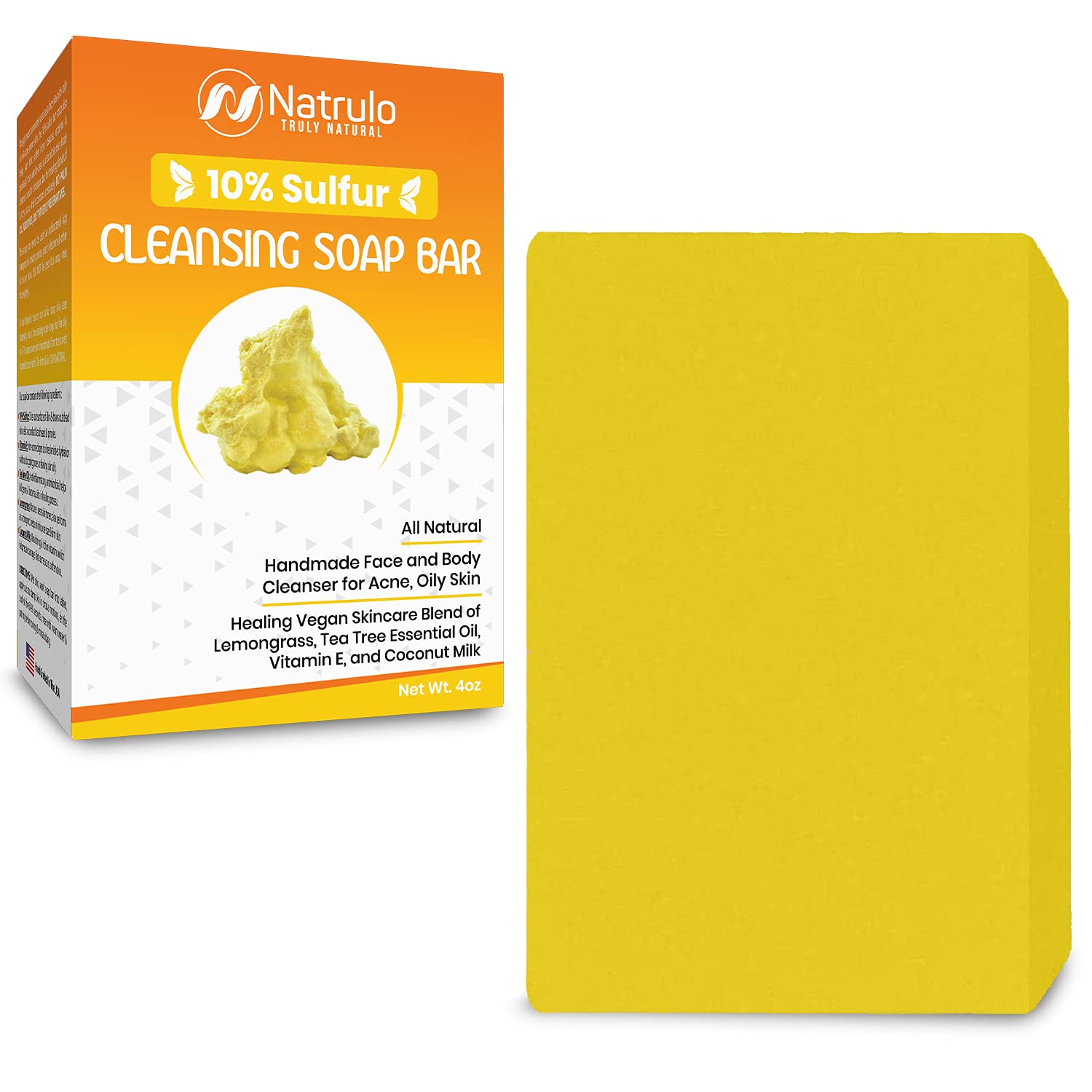This is an advertising photo for Natrulo's Cleansing Soap Bar. The product packaging has an ombre design with the top half transitioning from dark orange to yellow, and the bottom half is white featuring small gray triangles. The brand name "Natrulo" is prominently displayed at the top, followed by the text "Truly Natural" and "10% Sulfur." Below, a white circle showcases an image of the soap, depicted as a yellow blob. The box further describes the soap as an "All Natural, Handmade Face and Body Cleanser for Acne, Oily Skin, Healing Vegan Skincare Blend of Lemongrass, Tea Tree Essential Oil, Vitamin E, and Coconut Milk." The net weight of the soap is indicated as 4 ounces. The left side of the box contains additional text, though it is too small to read, and there is another image of the box on the right side, depicted entirely in yellow.